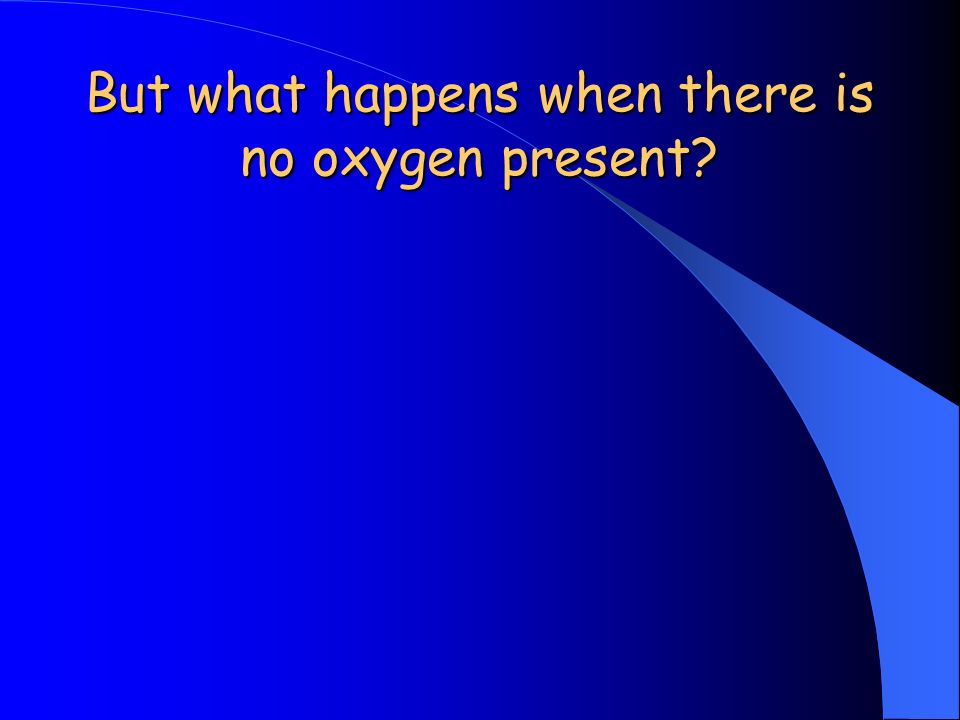This image appears to be a slide from a PowerPoint presentation featuring a predominantly blue background. The color gradient starts as a very bright blue on the left side and transitions to a darker blue, nearly black, in the upper right corner. A lighter blue pattern originates from the bottom right corner, gradually extending toward the upper left corner, becoming finer and more tapered as it ascends. The upper portion of the slide contains text in a mustard yellow, easy-to-read font that has a slightly childish appearance, reading: "But what happens when there is no oxygen present?" The text is situated primarily in the upper left section of the slide, leaving the center mostly empty. The yellow font may have a slight design element where a line runs between the words "present" and "happens." Overall, the slide suggests it is part of a sequence in a presentation, likely leading into more information or content below the current visible text.